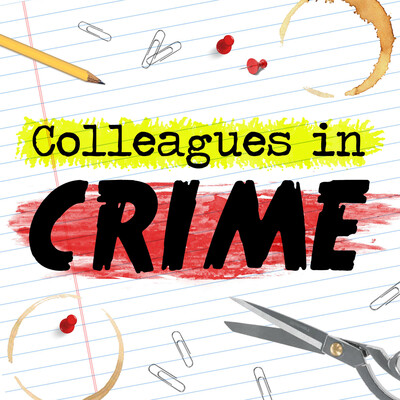The image is an intricate illustration of a piece of loose-leaf notebook paper with light blue lines and a red vertical margin, slightly angled to the left. Painted over the paper is the phrase "Colleagues in Crime," where "Colleagues in" is smaller, black text with a yellow background, and "Crime" is larger, black text against a red background. The word "Crime" is heavily emphasized and tilted around 30 degrees to the left. The paper is adorned with various office supplies: towards the upper section, there is a yellow pencil, several metallic paperclips, two red thumbtacks, and a circular coffee stain. The lower section of the paper features more thumbtacks and paperclips, with an additional coffee ring encircling a red tack. A partially open pair of silver scissors, appearing poised to cut through the letter "R" in "Crime," lies in the bottom right corner, angled upward toward the top left. The scene vividly captures a chaotic yet meticulously arranged desk setup.